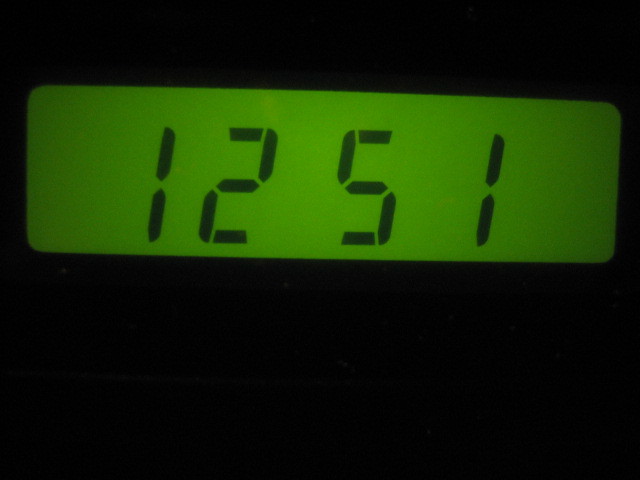The photograph showcases an up-close view of a digital display set against a pitch-black background, making it unclear what device the screen is a part of. Dominating the upper center portion of the image is a rounded neon green rectangle that spans much of the horizontal axis. Inside this illuminated rectangle, the black digits "1251" are prominently displayed, though they lack a colon, suggesting an unconventional time display. The digits are formed by segmented lines, reminiscent of a digital alarm clock or a calculator. Despite the ambiguity of the object, the picture depicts a focused and clear representation of the illuminated numerical display against the dark backdrop.